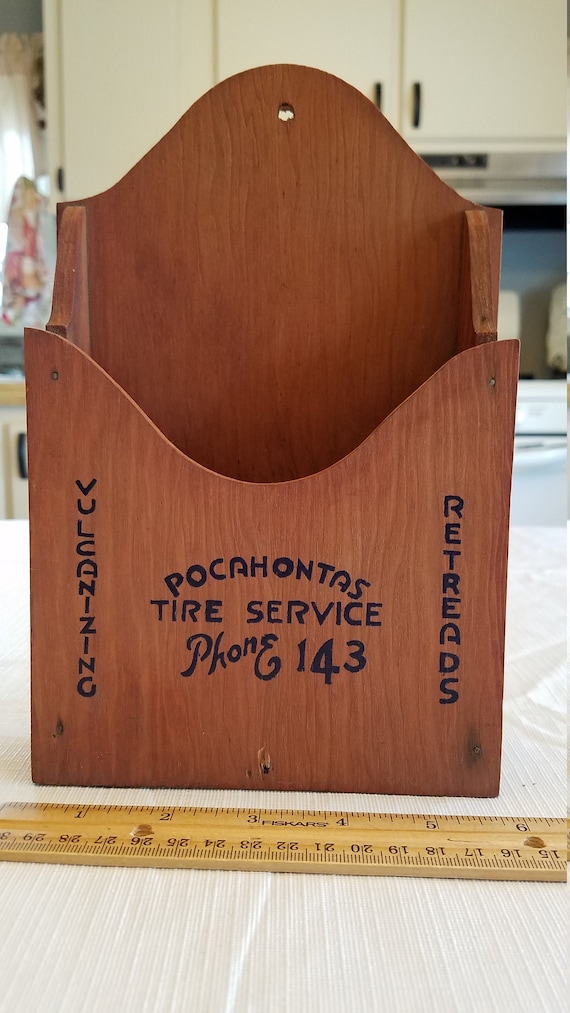The photograph captures a vintage, wooden mailbox-style holder, possibly for paperwork, situated in a kitchen setting. The rustic holder, resembling an old advertisement piece, is placed on a white plastic tablecloth with a textured pattern of lines. A light-colored wooden ruler with black numbers lies horizontally in front of the holder. The holder itself is made of unstained brown wood and features distinct curved edges both on the top back plate and sloping towards the center front. 

The front face of the holder is detailed with hand-painted text in black. On the left side, the vertical text reads "Vulcanizing," while the right side features the word "Retreads." In the center, the name "Pocahontas Tire Service" is prominently displayed with "Pocahontas" slightly arched and "Tire Service" horizontally aligned. Below this, in a stylized cursive, it reads "Phone 143." The holder also features small nails visible on the corners and face.

In the background, a beige countertop and cabinets, a stainless steel range hood, and a white stove are visible. To the left, a kitchen window framed with a white curtain and a dishrag hanging on the side of the cabinets can be seen, highlighting the domestic setting of the scene.